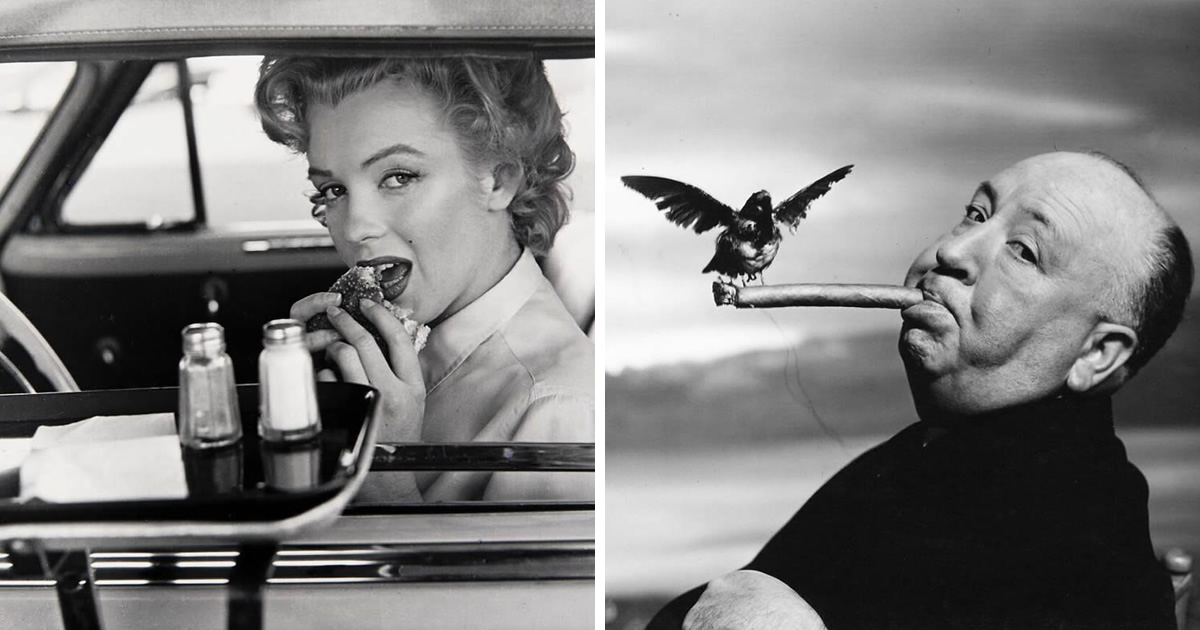The black-and-white image is divided into two distinct square photographs. On the left, Marilyn Monroe is captured sitting in a car reminiscent of a drive-in restaurant. She is in mid-bite of a sandwich, her mouth open as she looks towards the camera. A tray hangs from her car door window holding what appear to be salt and pepper shakers and a white napkin. On the right, Alfred Hitchcock is depicted leaning back with a cigar in his mouth. At the edge of the cigar, a bird perches with its wings outstretched. Both photographs are very clear and bathed in natural light.